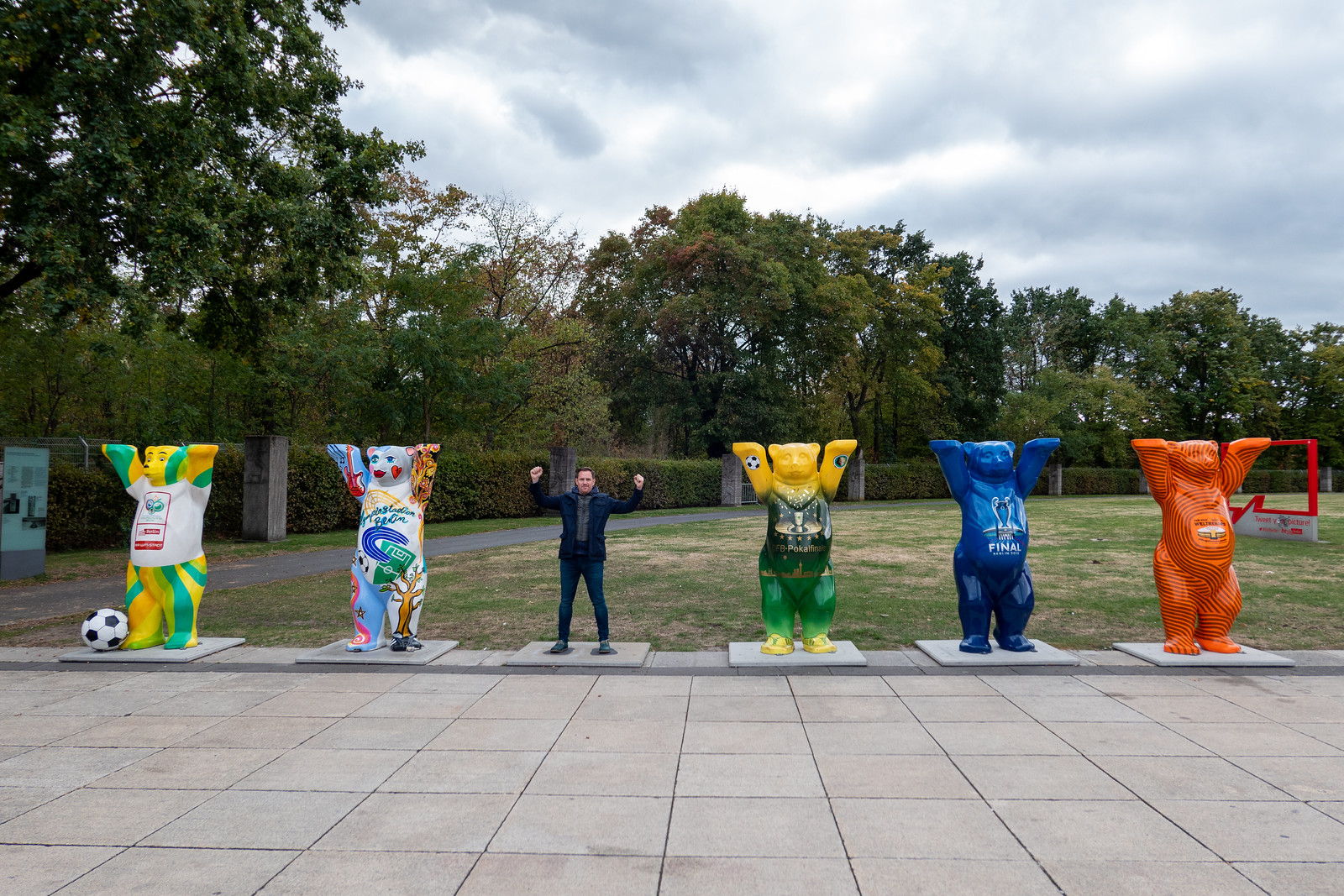In an outdoor scene featuring mascots, the photograph captures a slightly overcast sky with clouds in the distance. Prominent is a hedge wall stretching from left to right, behind which a line of tall, green trees can be seen. A stone-tile walkway extends across the scene. On this walkway, there are five colorful mascot statues and one human, all with their hands raised in the air. The mascots are vibrant and varied: a blue and green one with a white shirt and a black and white soccer ball, a partly white and light blue bear with red accents, a green mascot that transitions to gray and then yellow, an all-blue mascot, and an all-orange one. Among them stands a human dressed in a dark blue outfit, mimicking the mascots with arms held high. At the bottom of the scene is a grassy field, adding a natural touch, while the background is framed by the distant clouds above the trees.